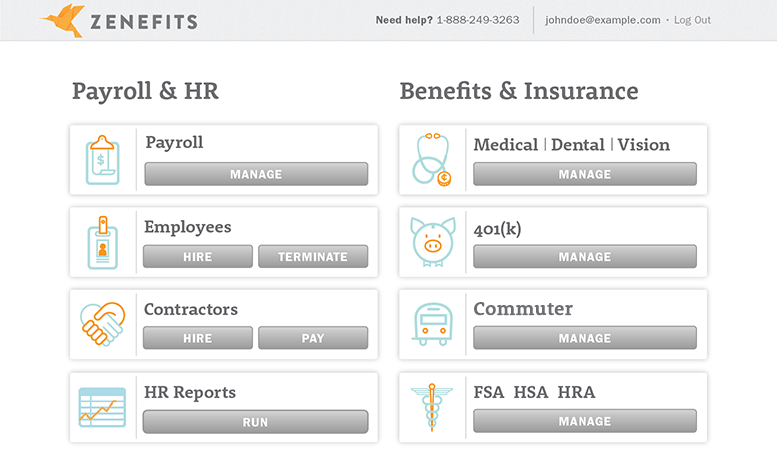In the upper left-hand corner of the webpage, there is an orange bird logo adjacent to the word "Zenefits," spelled in large, block, and capitalized letters. Immediately to the right of "Zenefits," the text reads: "Need Help? 1-888-249-3263." Following this, a small vertical gray line separates the contact information from the user's email, "John Doe at example.com," which is further to the right and followed by a light gray "Logout" link.

The main webpage layout is divided into two primary columns. The left column focuses mainly on Payroll and HR management, featuring the following sections:

- "Payroll," which offers payroll management functionalities.
- "Employees," which includes buttons for "Hire" and "Terminate."
- "Contractors," which includes buttons for "Hire" and "Pay."
- "HR Reports," which has a "Run" button.

The right column is dedicated to managing benefits and insurance, with several sections listed as follows:

- "Benefits and Insurance," under which "Medical," "Dental," and "Vision" options are found, each accompanied by a "Manage" button.
- "401K," which also provides a "Manage" button.
- "Commuter," featuring a "Manage" button.
- "FSA, HSA, HRA," accompanied by a single "Manage" button for these flexible spending accounts.

The webpage is designed for easy navigation and management of various payroll and HR functions, offering a comprehensive overview for administrators and users.